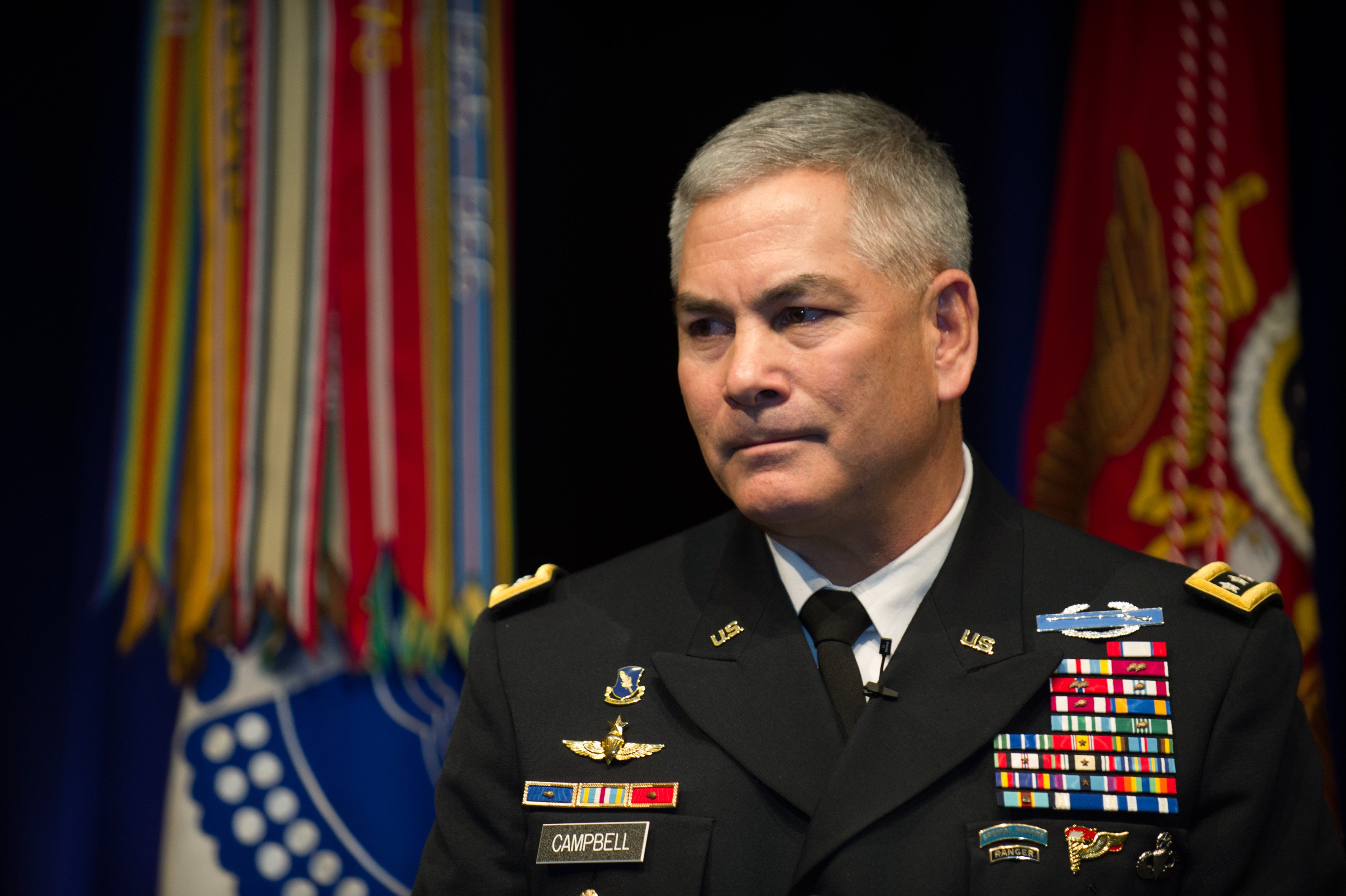The image depicts a distinguished military officer, identified by the name "Campbell" on his jacket. He is wearing a formal black coat adorned with significant insignia. The coat features a high-collared design with "U.S." and gold embellishments on both sides of the collar. On his lapels, three prominent gold stars indicate his high rank. His attire includes a crisp white shirt and a black tie.

The left side of his chest displays a blue pin with a white horseshoe alongside an impressive nine rows of colorful service ribbons, symbolizing various achievements and honors. Below these ribbons, there are three additional military pins. The right side of his coat also features another set of service bars and two more pins above them. His name tag, "Campbell," is prominently placed.

Campbell's expression is serious and contemplative as he gazes to the left, and his gray hair is neatly trimmed. The background is predominantly dark, suggesting an indoor setting, possibly at a podium or formal event. Behind him, a series of vibrant flags provide a stark contrast to the dark background. To his left, there is an array of flags in yellow, blue, red, and white colors, creating a striking and colorful display. On his right, a red flag with yellow accents is visible. The overall ambiance conveys a sense of solemnity and honor.